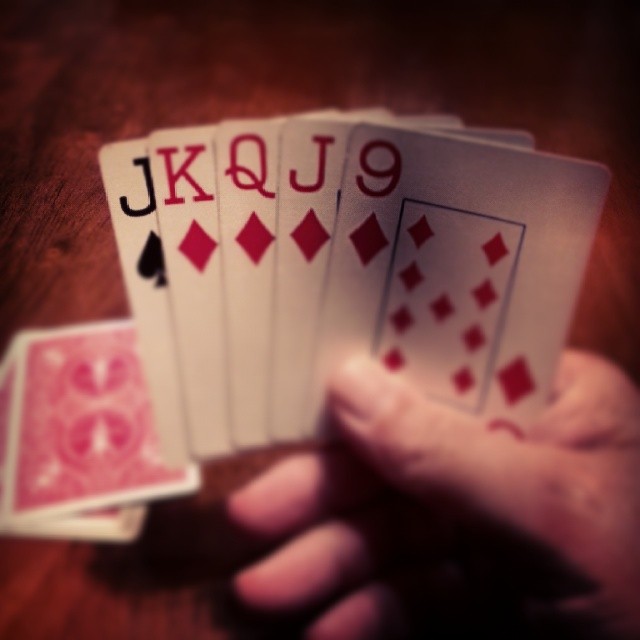This photograph captures a close-up view of a hand of cards being played on a brown, wood-colored table. The perspective is from the person holding the cards, a Caucasian male, and shows no other players or cards. The deck is placed face-down on the table. In the hand, there are five cards: a Jack of Spades, a Jack of Diamonds, a Queen of Diamonds, a King of Diamonds, and a Nine of Diamonds. The player is just a Ten and an Ace of Diamonds away from forming a royal flush. The cards feature red ranks for diamonds and black for spades, with white backgrounds and red-and-white patterned backs. The table, though not real wood, appears wood-like in color and texture, adding a rustic feel to the scene.